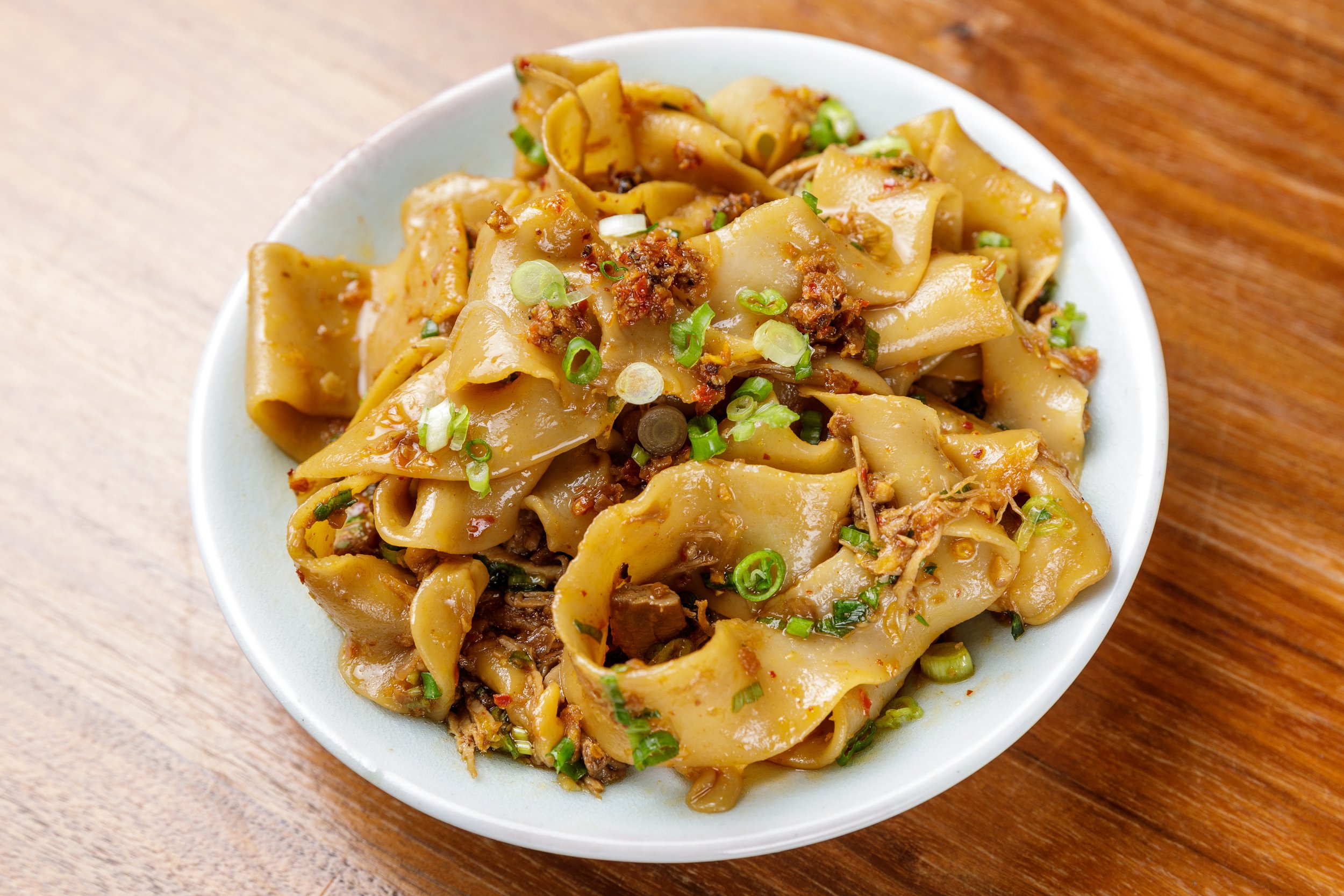The photograph captures a top-down view of a dish placed on a flat, white plate, likely made of plastic or ceramic. The dish predominantly features glossy, fresh pasta with a wavy texture, indicative of its Asian, possibly Chinese, inspiration. Interspersed within the pasta are bits of meat, varying in color from brown to reddish, and adorned with green vegetables that appear to be scallions or spring onions. The plate rests on a richly marbled wooden table, characterized by a deep brown hue with darker brown patterns, adding a rustic contrast to the vibrant and detailed dish. The overall appearance suggests that the pasta might be spicy, given its visual presentation and the ingredients observed.